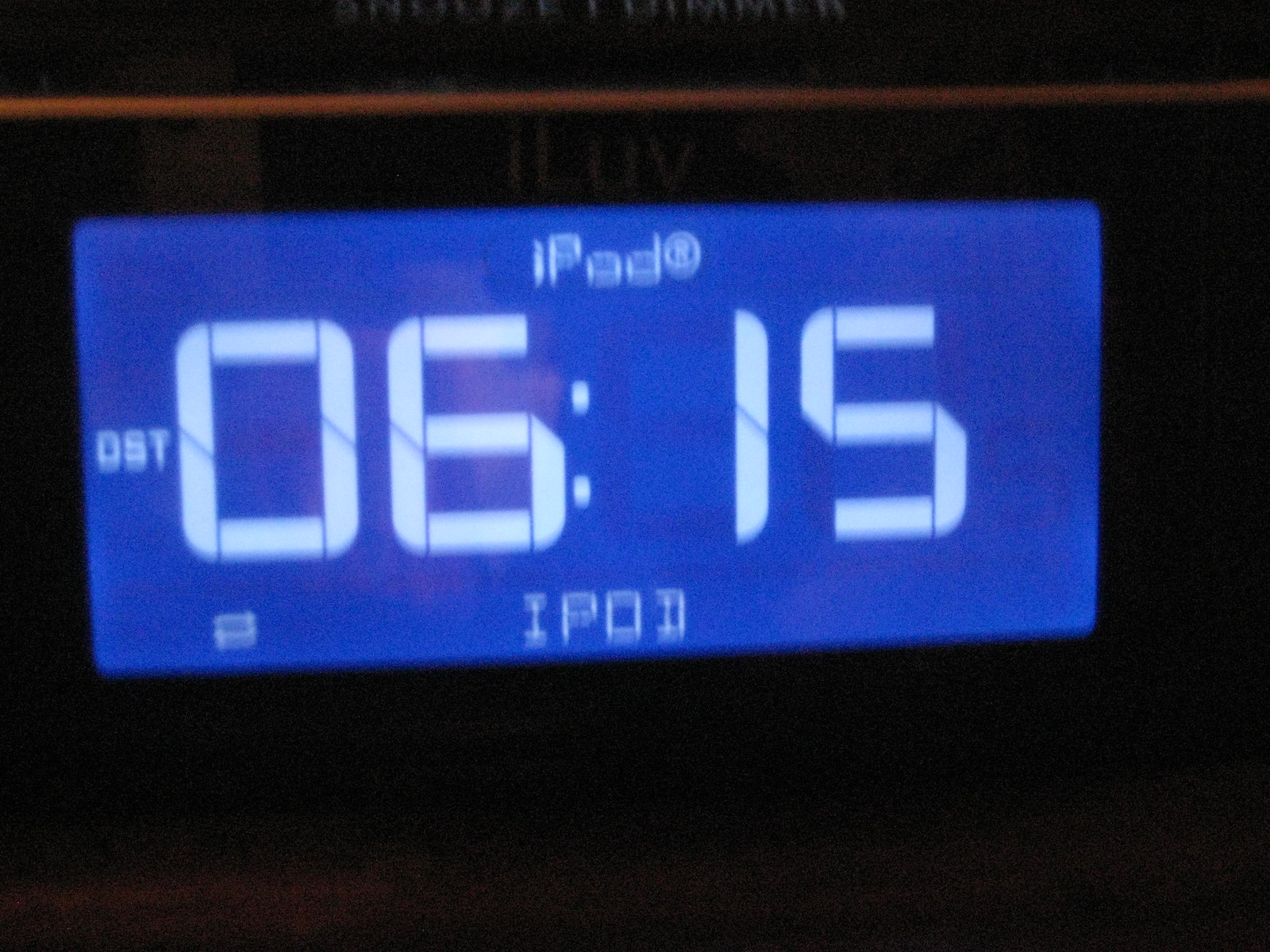This low-resolution, square-shaped image is blurred and pixelated, with the top and bottom sections fading into blackness. Dominating the center is a digital screen, the clarity of which stands out against the indistinct background. Across the image from left to right runs a faint, orange line, its exact nature difficult to discern due to the poor image quality. The screen itself is blue, displaying white text. At the top, it reads "iPod," followed by "OST06:15," and then repeats "iPod" once more below. The overall image quality makes it challenging to identify finer details.